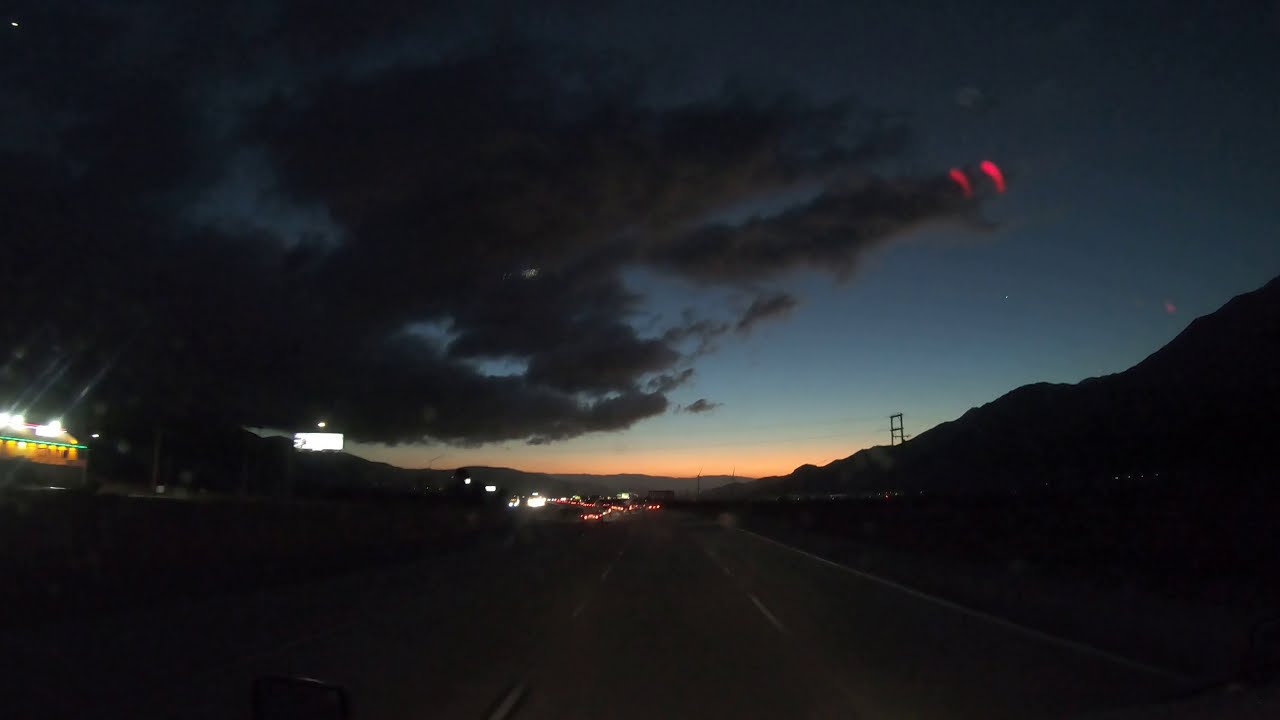This vibrant, full-color photograph captures the serene moments just after sunset. The deep night sky transitions from a profound dark blue at the top down to a lighter blue and ultimately a soft, peachy glow near the horizon. Dark clouds dominate the sky, interspersed with faint hints of red, possibly reflections from distant lights. 

Taken from the perspective of a vehicle—likely a motorcycle or car due to the visible side view mirror and windshield reflections—the image provides a fascinating urban-rural contrast. On the far left, a brightly lit yellow building with a green awning stands out against the twilight. In the middle and stretching into the distance, the taillights of numerous vehicles illuminate a three-lane road, suggesting bustling activity even at this hour. 

To the right, rolling hills and a prominent electrical tower are silhouetted against the gradually lightening sky. The beauty of this scene is enriched by the presence of subtle red hues in the clouds, adding depth and complexity to the composition. Overall, the photograph captivates with its blend of natural and man-made elements, set in the tranquility of post-sunset glow.